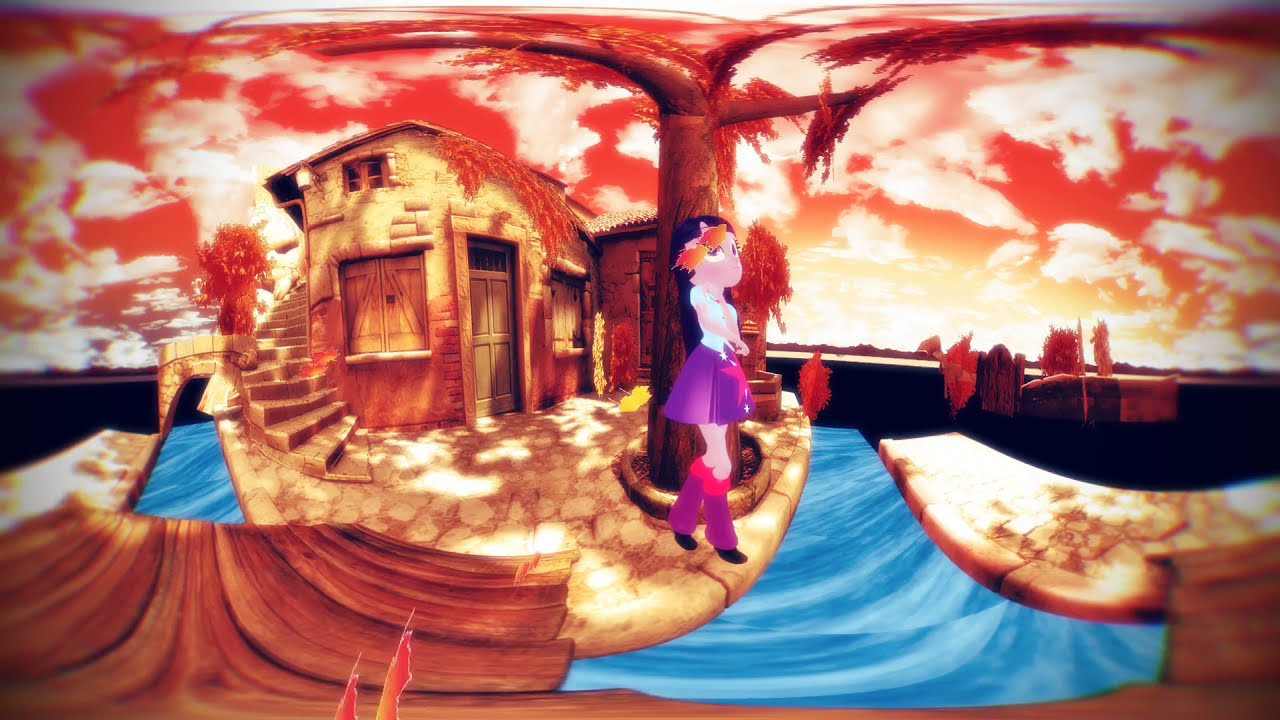In this vivid animated artwork, a teenage girl with waist-length black hair, adorned with what might be an orange and yellow bow or streaks of dyed hair, stands prominently. She is dressed in a white short-sleeved shirt and a purple skirt with a possible star detail, paired with purple leggings or leg warmers and black shoes. The girl is gazing up at a sky rendered in dramatic shades of orangish-red transitioning to yellow-orange, filled with surreal clouds. Behind her, a quaint, stone house features a winding staircase that wraps around its structure, with a flowing half-circle of water and a bridge nearby. The scene is further characterized by a stark tree with bare branches emerging from a stone enclosure and flanked by red-tinged trees, enhancing the fantastical and whimsical nature of the landscape.